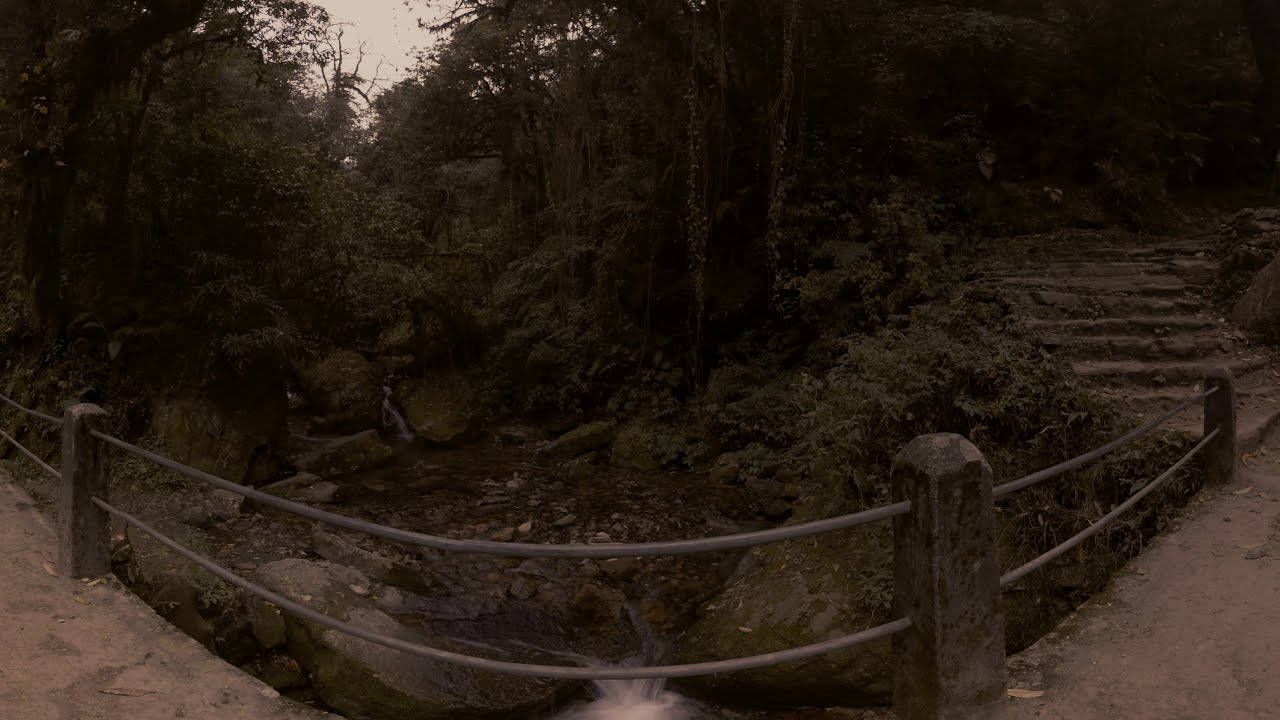This detailed panoramic photograph captures a serene hiking trail within a lush forest, presented with a fisheye-like distortion that curves the image. The dirt path, flat at certain points, transitions into rocky stairs that ascend into the dense woods on the right. Flanked by a metallic railing interspaced with thick stone posts, the trail overlooks a shallow ravine featuring a sparse water stream coursing through a bed of rocks. Tall green trees and various plants grow densely on either side of the stream. Additionally, there's a modest rope fence enhancing the path's rustic appeal. The sky, appearing white with a slight pinkish hue, suggests an overcast day or the onset of dusk, casting a dim and tranquil light over the scene.